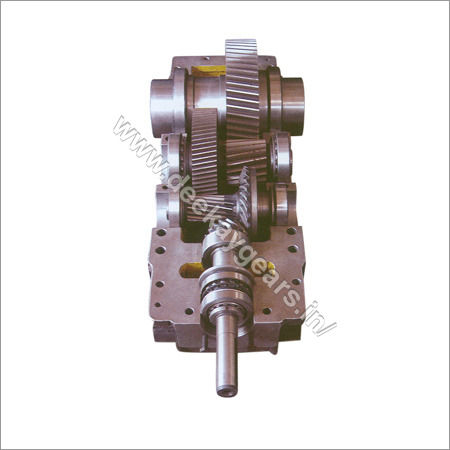The image features a substantial piece of machinery, specifically a large mechanical gear, primarily constructed of silver-gray metal with hints of yellow in the grooves. The gear's sharp, interlocking teeth suggest a robust design intended for heavy-duty applications, possibly in aviation or automotive vehicles. A metal rod is prominently positioned, facing the viewer, indicating it as an integral part of the gear's mechanism. The object is isolated against a plain white background, with no other elements present. A watermark displaying the URL "www.dkgears.in/" spans diagonally across the gear, highlighting the manufacturer's website, spelled out as D-E-E-K-A-Y-G-E-A-R-S. The gear, which appears to need lubrication for optimal performance, conveys a sense of weight and durability, though it’s not excessively large in scale.